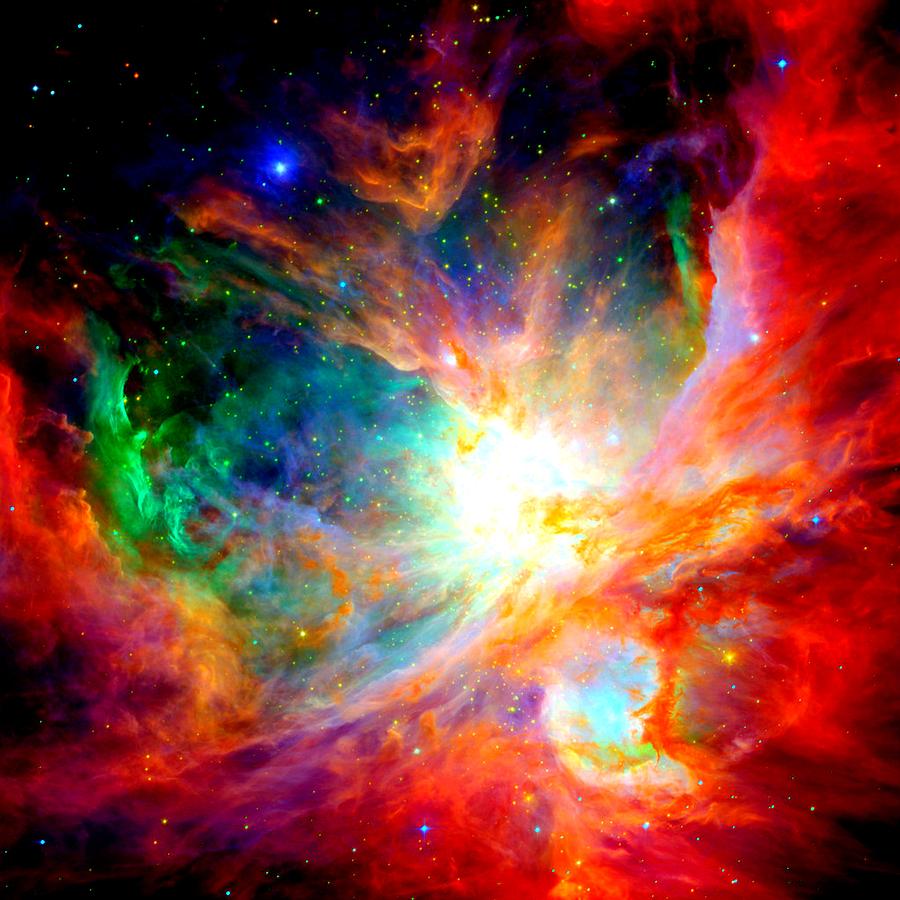The image depicts an ethereal cosmic scene, possibly a digitally rendered depiction of a nebula in deep space. It features an intricate blend of vibrant colors, ranging from burning reds, yellows, and oranges at the foreground to cooler hues like blues, greens, and purples towards the background. At the center, a luminous white light source stands out, radiating an intense glow that illuminates the surrounding nebula. This light transitions into various vivid shades creating a tie-dye-like pattern, with the left side of the image predominantly showcasing green and blue tones. Scattered throughout the dark, star-studded background, twinkling stars add depth and a sense of the vast expanse of the universe. The entire composition creates a stunning display reminiscent of a distant galaxy, highlighting the boundless beauty and mystery of the cosmos.